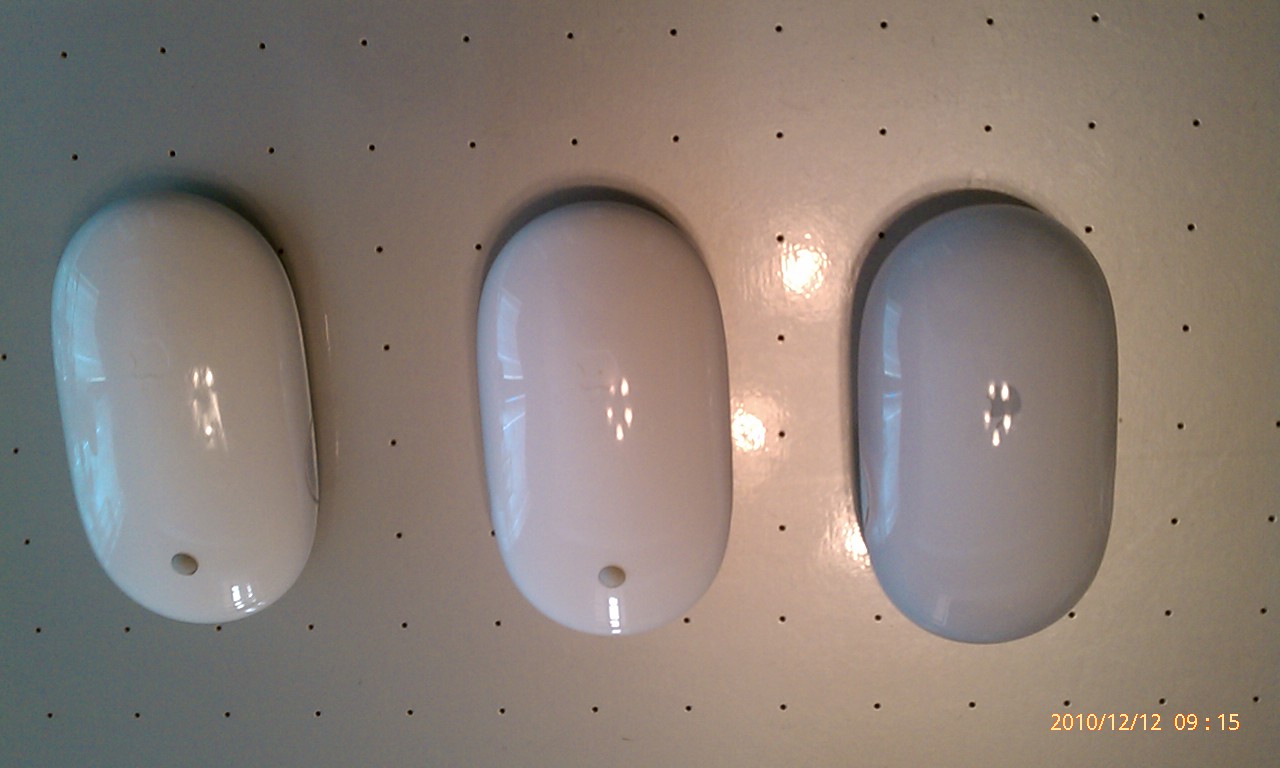The photograph, taken on December 12, 2010 at 09:15 as indicated by the orange timestamp in the bottom right corner, features three Apple computer mice aligned horizontally on a light beige metal surface perforated with equally spaced pinholes. The mice, resembling rounded ovals much like bars of soap, are positioned with their long axes running up to down. They are not equally spaced, with the middle and right mice slightly closer together. The colors of the mice vary due to lighting and possibly image tonality: the one in the center is the most piercing white, while the left one is slightly off-white and the right one appears almost grey. Each mouse has a discernible grey track wheel, with small, barely visible Apple logos on them. Reflections from lights can be seen between the two rightmost mice, adding to the overall glossy appearance of the mice against the grey-toned background.